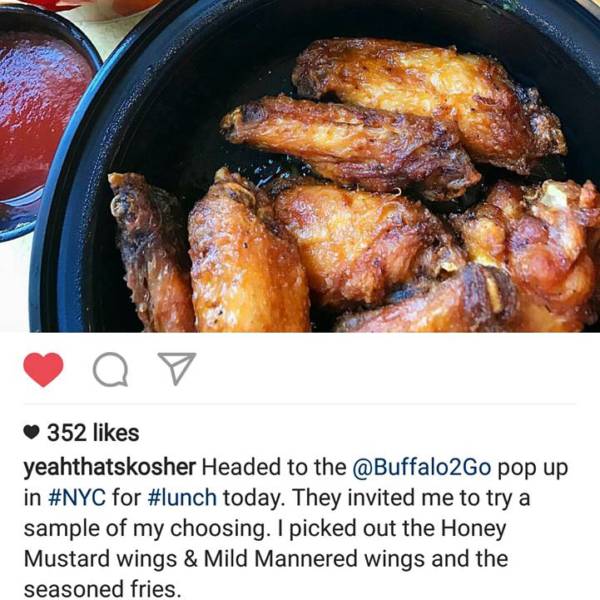In this Instagram post, a delectable spread is showcased: a black pot brimming with seven crispy, golden-brown chicken wings sits prominently in the center. To the upper left, a smaller black bowl contains a vibrant red marinara sauce. The post is set against a clean, white table background, providing a stark contrast that enhances the food's visual appeal. Above the main image, a sliver of a red pot is barely visible. Below the image, Instagram graphics are displayed: a red heart indicating "352 likes," a white speech bubble for comments, and a white paper airplane for sharing. The text below reads, "Yeah, that's kosher! Headed to the @BuffaloToGo pop-up in #NYC for #lunch today. They invited me to try a sample of my choosing: honey mustard wings, mild-mannered wings, and seasoned fries."